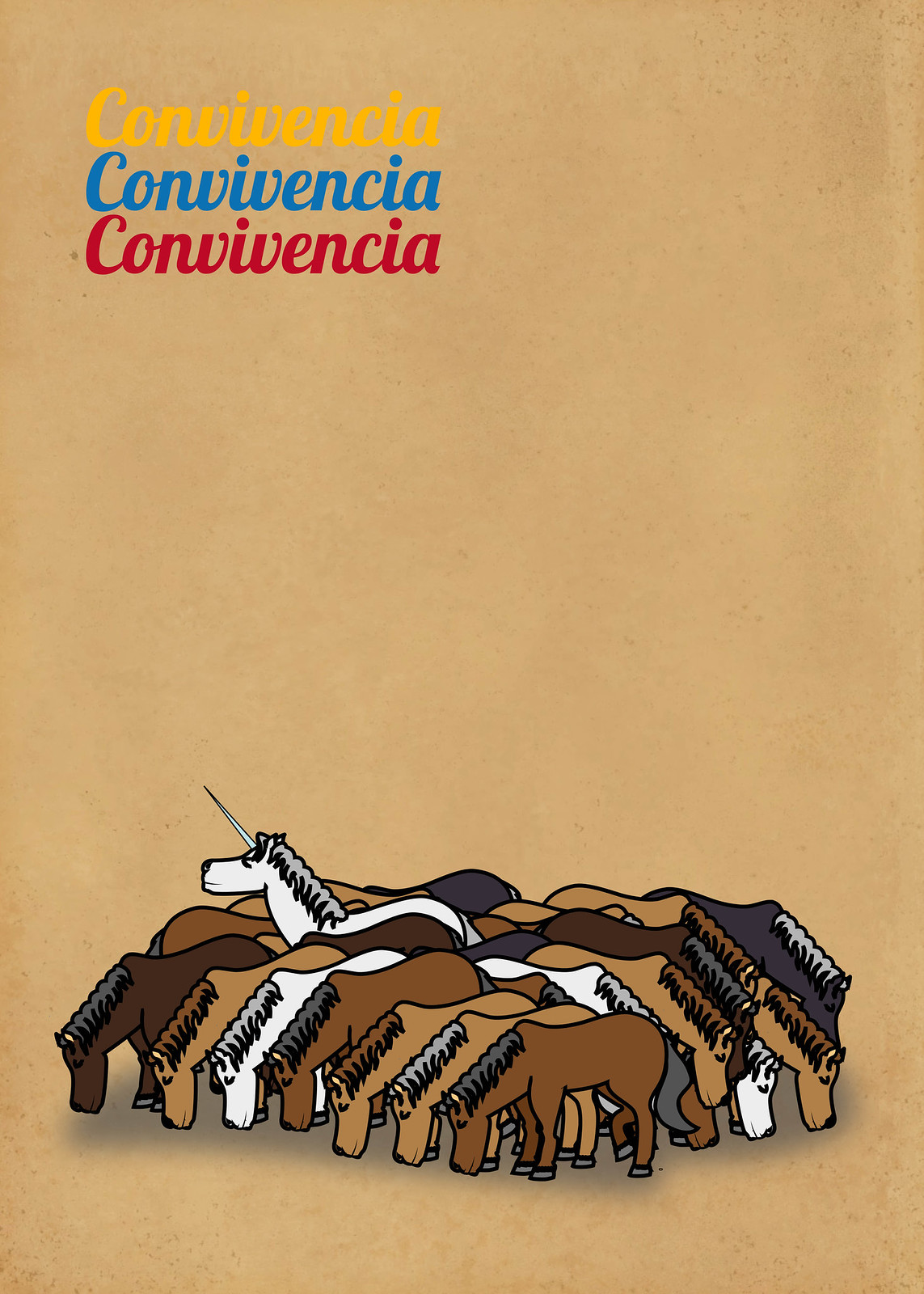The image is a vertically-oriented, brown poster resembling the color of a paper bag, measuring approximately six inches tall by four inches wide. In the upper left-hand corner, the word "Convivencia" is repeated three times in cursive script, written in gold yellow, blue, and red. Below the text, a herd of cartoon horses with varying colors—dark brown, light brown, very pale tan, gray, and white—are shown with their heads down, appearing to graze on grass. Among these identical horses, one distinct figure stands out: a white unicorn with a large turquoise horn, its head raised and looking to the left, in contrast to the feeding horses.